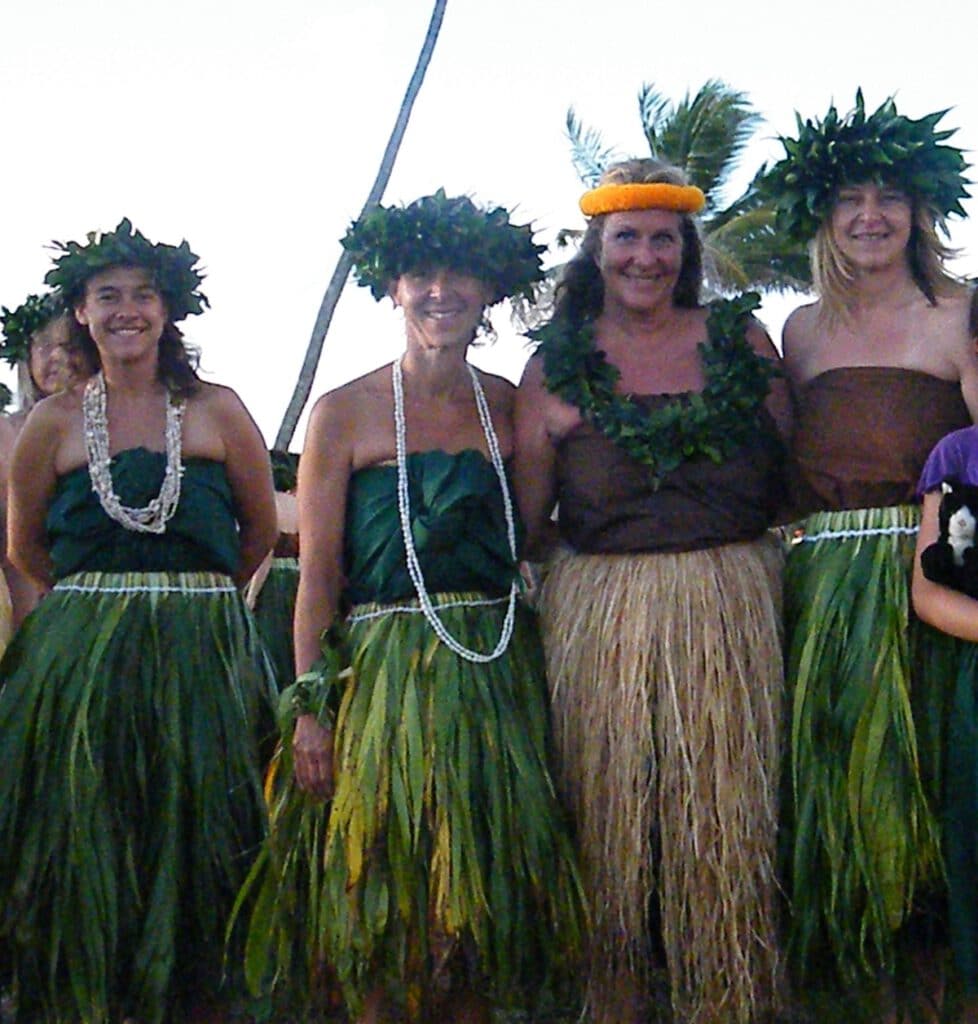In this photograph, four women stand side by side, each dressed in Hawaiian-style costumes that feature sleeveless tops and long grass skirts. Three of the women wear green garlands on their heads, while one dons an orange headband. Two women sport white necklaces, another has a green garland as a necklace. The tops consist of green and brown hues, with two women in green tops and the other two in brown. The grass skirts vary in color: three are green and one is light brown, resembling straw. Their hair, either long or tied up, ranges from brown to white. The women appear cheerful and are either of a tan or pale complexion, suggesting a mix of ethnic backgrounds. Behind them, a palm tree can be seen against a white sky. To the left, there is a partial figure of another woman, and to the right, a glimpse of what seems to be a child holding a stuffed animal, possibly a black cat. This image captures a likely Hawaiian or Native celebration, filled with joyous expressions and cultural attire.